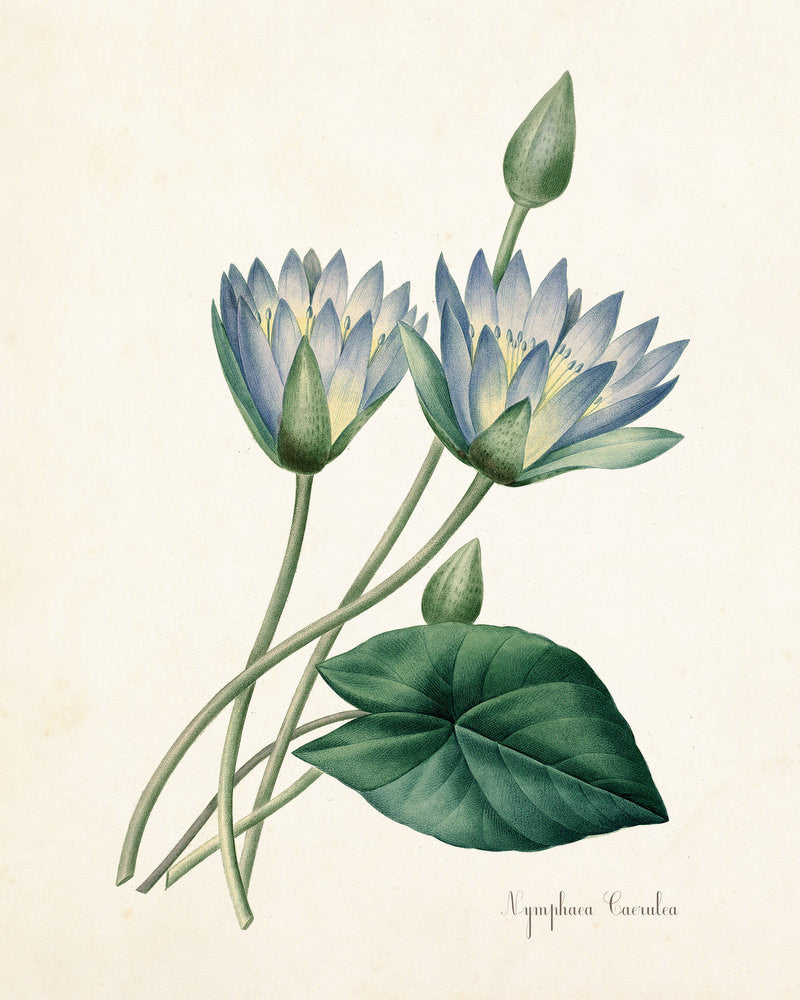This detailed illustration features a cream-colored, aged-looking background, evoking the feel of an old botanical print. Dominating the scene are blue-petaled flowers with distinctive yellow centers, showing varying stages of bloom. Two central flowers are in full bloom, displaying their intricate, elongated petals, while adjacent buds, still unopened, hint at impending blossoming. The flowers are supported by thin green stems, and lush green leaves form a striking contrast, including a prominent, large leaf folded sideways at the bottom of the image. The botanical name "Nymphaea caerulea" is elegantly inscribed at the bottom in dark, cursive font, identifying this water lily species. The illustration merges artistry with scientific precision, offering a glimpse into the delicate beauty of this aquatic plant.